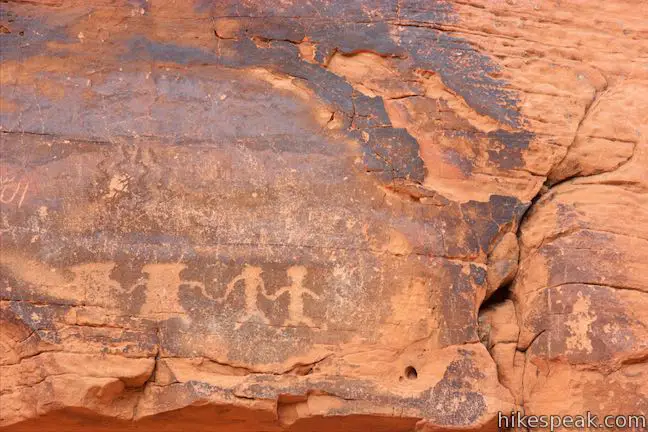The photograph showcases an ancient rock adorned with cave writings, horizontally framed in a rectangular format. The bottom section of the image bears the website watermark "HIKEPEAK.COM." The stone itself exhibits a striking peachy-pink hue across various sections, transitioning into brown and darker brown areas covering roughly half to two-thirds of its surface. The focal point of the image lies in the intricate carvings on the lower left-hand side of the stone, depicting a fascinating scene. The carvings include two cylindrical figures with small protruding shapes at both the top and bottom, resembling lips. These figures each have two hands and their legs splayed outward. They are interconnected by holding hands in a chain with two additional figures. These additional figures resemble stick people, but with slightly thicker bodies, circular filled-in heads, and extended arms. Together, the four figures form a chain, all holding hands and spreading their legs in unison, capturing a moment of ancient artistry and cultural expression.